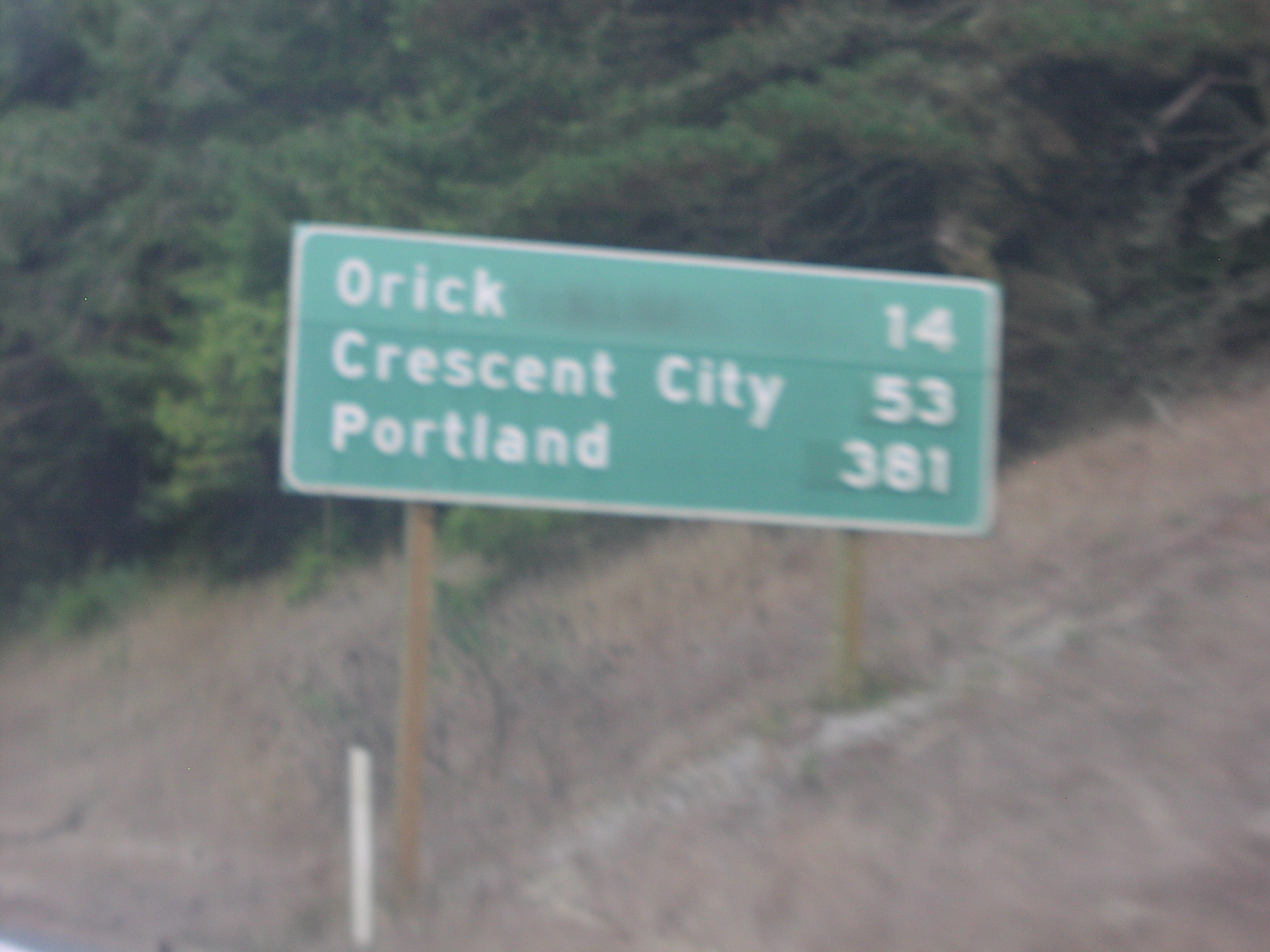This photograph depicts a rectangular green road sign with white text, mounted on two wooden posts of different heights, situated on a hill that rises from left to right. The sign indicates distances to three cities: Orick (14 miles), Crescent City (53 miles), and Portland (381 miles). In the background, dense evergreen trees and greenery are visible, suggesting a west coast location. In front of the sign, the ground is covered with dry, brown grass and weeds, and a short white post stands to the left of the sign. The image appears to be taken during the day, though it is low resolution and the lighting suggests an overcast sky, dawn, or dusk.